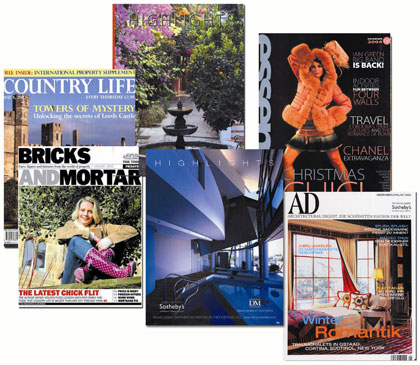The image depicts a visually rich assortment of six commercial home-related magazines, some overlapping but all partially visible, arranged on an assumed coffee table setting. The titles include "Country Life," "Bricks and Mortar," "Highlight," and "A.D." The cover of "Bricks and Mortar" is nearly fully visible and features a woman sitting on a chair with purple boots. "Country Life" showcases a blue sky and a castle with the headline "Towers of Mystery." The magazine titled "Highlight" is in the center of the collection, showing a bluish interior scene, likely an indoor pool with cool blue lighting. Another cover has the word "Christmas" and features a woman adorned in a large, bear-like brown scarf, enveloping her head and extending down to her waist. One magazine cover is mostly obscured but appears to depict lush garden foliage, while "A.D." presents a serene bedroom interior with a prominent window. The vibrant colors span from bright oranges and pinks to calming blues and greens, creating a collage of visual interest and thematic diversity centered around home and lifestyle.